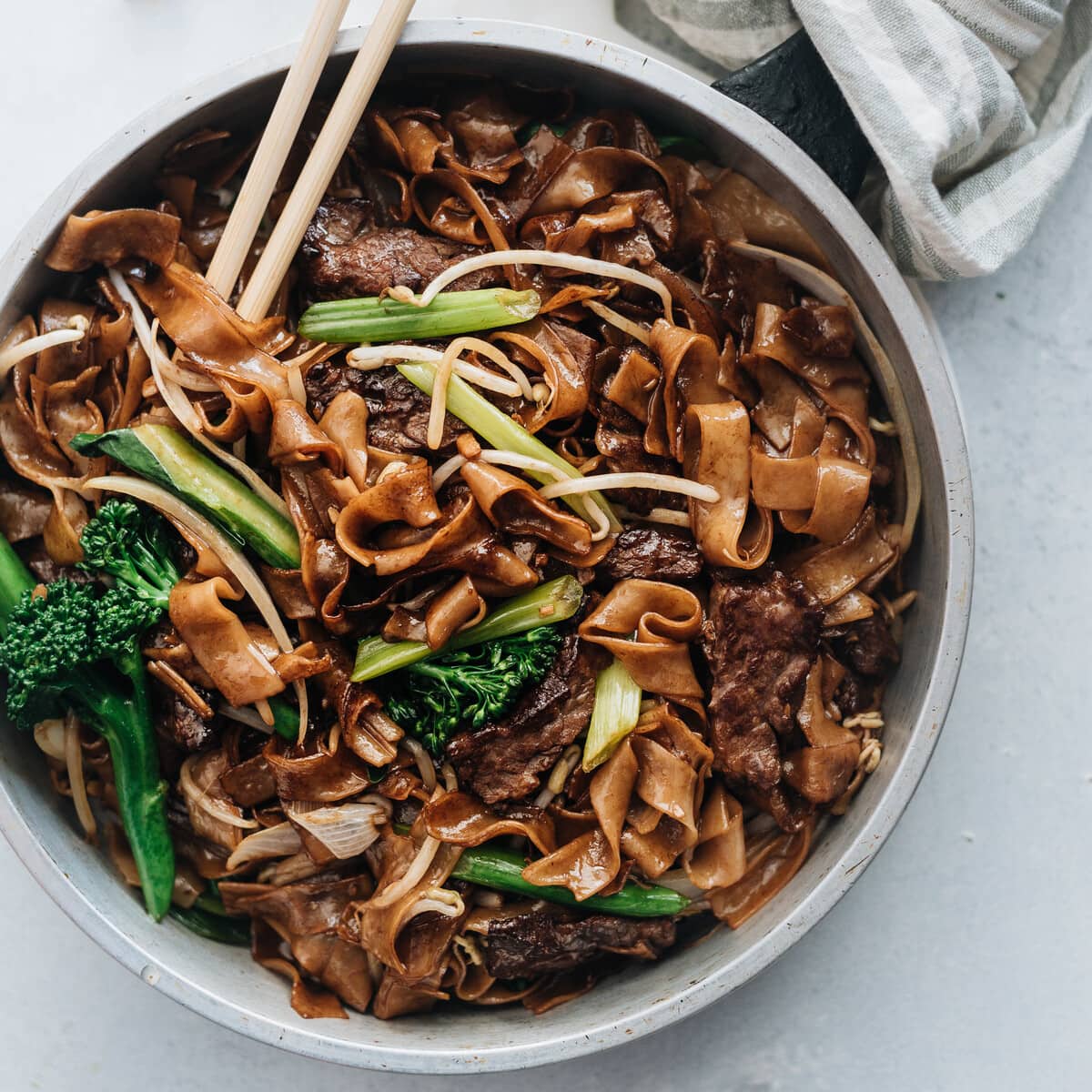The image features a close-up of a vibrant noodle dish, likely Asian in origin, possibly Thai or Cantonese. The food is presented in a speckled white and gray bowl that sits on an off-white surface with grayish hues, resembling granite. A black handle peeks out from underneath a gray and white cloth napkin at the top right. The dish is a savory mix of dark brown noodles, possibly stir-fried, coated in a rich, brown sauce. Dark-colored meat, which could be beef, intertwines with the noodles. The bowl is garnished with fresh green vegetables, including large chunks of Chinese broccoli, celery, and green beans, mostly congregated on the left side of the bowl. Chopsticks are positioned at the top left of the bowl, adding an authentic touch to the delicious and juicy presentation.